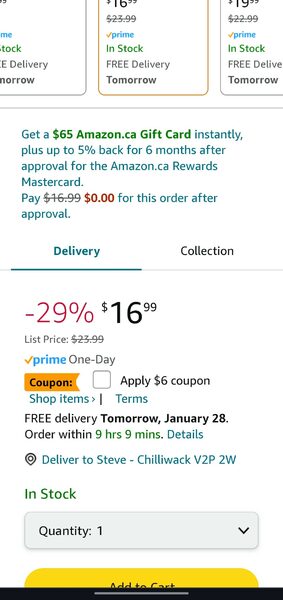Title: Amazon.ca Page Details with Prime Offers and Promotions

Description:
The image captures a detailed section of an Amazon.ca page, specifically a vertical rectangular segment. At the top, there are three partially visible items indicating their availability. Each item showcases the Prime logo in turquoise accompanied by a gold checkmark, with "In Stock" noted in green below, followed by "Free Delivery" and the promise of delivery "Tomorrow."

Below these items, a promotional message is written in blue-green text offering a "$65 Amazon.ca gift card instantly", alongside up to "5% back for six months" upon approval for the Amazon.ca Rewards Mastercard. The offer details also clarify that a $16.99 fee is waived, showing "0.00" in orange for the order after approval.

The mid-section features two columns; the first labeled "Delivery" in blue-green text, and the second labeled "Collection" in black with a red discount notation of "-29%," alongside a black "$16.99" price. The original list price of $23.99 is crossed out in light gray. Both columns include the Prime logo in turquoise next to "One-day" delivery in gray.

Further down, there is a coupon section with the word "Coupon" in an orange rectangle with black text, followed by a blank square to "Apply $6 coupon" written in black. Next to this is a button labeled "Shop Items" in turquoise with "Terms" on the opposite side.

A section promises "Free Delivery" in black, with "Tomorrow, January 28th" in bold black text. Details about the ordering timeframe follow, with "Order within" in black and "9 hours, 9 minutes" in green. The delivery address is specified in turquoise: "Steve-Chilliwack, V2P2W." A prominent "In Stock" status is indicated in green beneath it.

At the bottom is a horizontally oriented light background with "Quantity 1" in black along with a down arrow for selection. Additionally, a yellow oval button displaying "Answer Card" in black is partially cut off by a black horizontal area at the bottom of the screen.